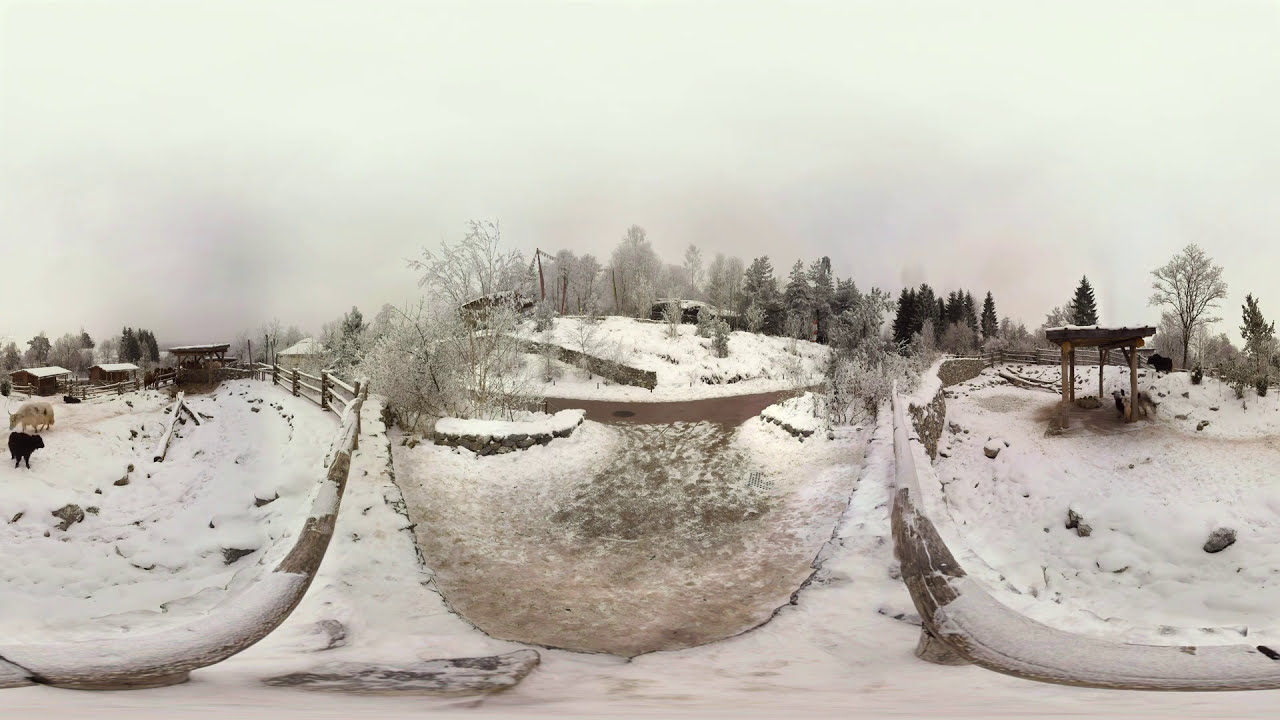This panoramic 360-degree image, captured with a fisheye lens, presents a winter scene of a snow-covered farm. The entire image is warped and flattened, creating a warped view of the landscape. Farm structures, which look rather insubstantial, appear on both the left and right sides—these might be simple open-sided shelters for the animals. The left side shows some animals in an enclosed area that looks partly wooden and partly stone. Among them is a sheep and possibly a calf or a humped bull. On the right, a cow is seen laying down.

In the foreground, shrubs, bushes, and bare trees are visible below a gray, overcast sky that blends seamlessly with the snow-covered ground, creating a very white, monochrome effect. There's also a hill with a walking path that curves up, bordered by what looks like a small fence. Power lines are visible in the middle of the image, stretching across the tree line in the background. This intricate depiction amalgamates all repeated and shared elements from the individual descriptions into one cohesive and detailed caption.